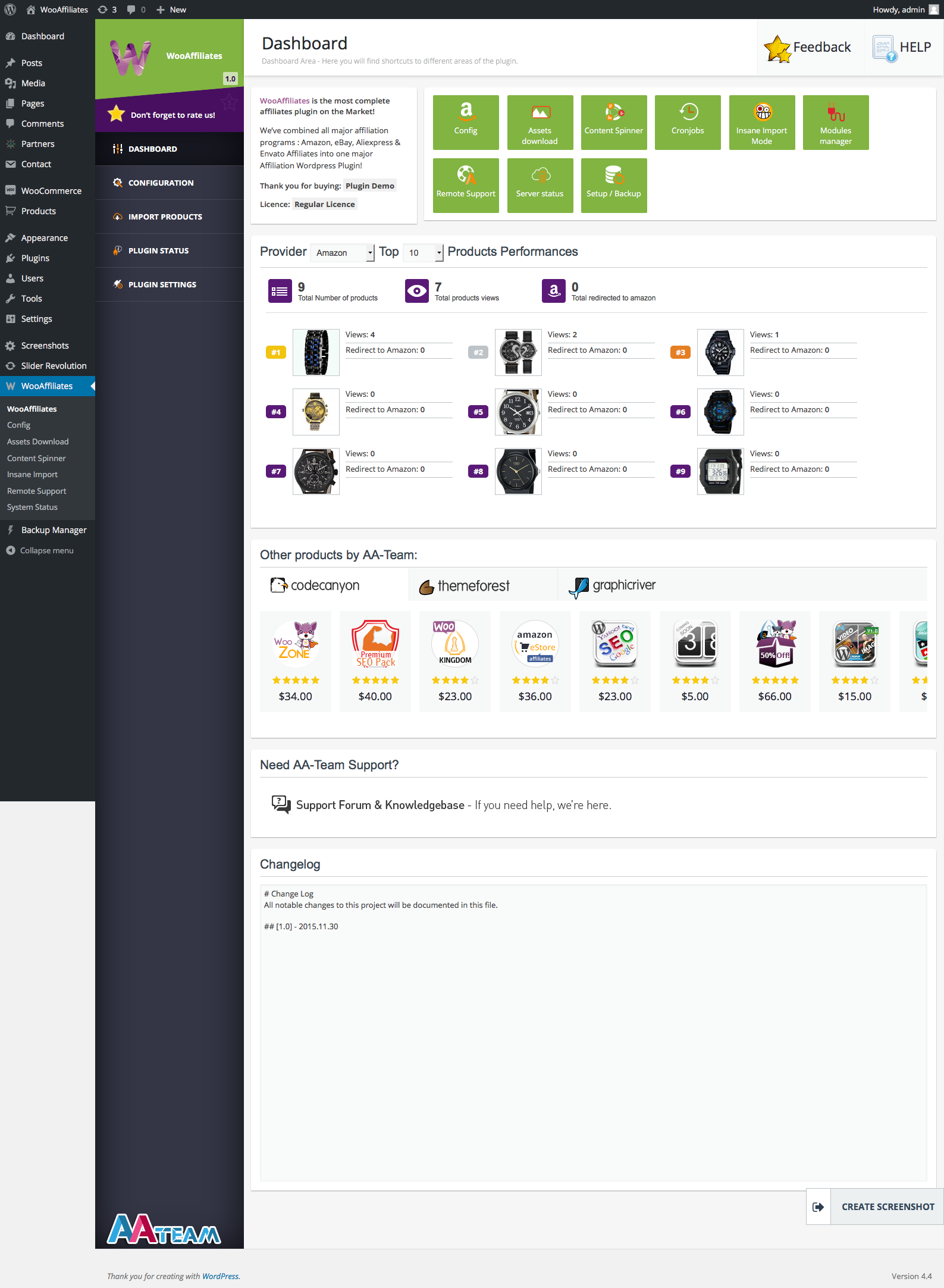Screenshot of a WooCommerce Admin Dashboard:
The image is a screenshot of an admin dashboard from a WooCommerce website, displayed in a profile orientation. The interface consists of two main rectangular sections, one nested within the other. 

In the upper section, we see a horizontal menu bar featuring several icons. On the top-right corner, a greeting message "Howdy Admin" is visible. On the top-left corner, a circular icon with the letter "W" is displayed next to the text "Woo Affiliates," accompanied by additional icons.

Beneath this, the main left-hand sidebar menu includes various options such as Dashboard, Posts, Media, Pages, Comments, Partners, and approximately 30 other clickable buttons or options. The "Woo Affiliates" section, about two-thirds of the way down this column, is currently selected and highlighted in blue.

The primary content area to the right displays the Woo Affiliates dashboard. Here, another menu appears on the left side, listing options like Dashboard, Configuration, Import Products, among others. At the top-right corner of this section, the word "Dashboard" is visible, indicating the main focus of the page. 

The content area provides an overview of the e-commerce site's performance, featuring details about products, performance metrics, and images of several products. Additionally, there are sections mentioning other products developed by AAT, further product images, and a section on support. The screenshot captures the structured layout and the comprehensive tools available for managing an e-commerce platform.